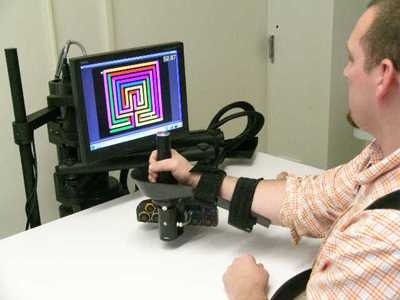The photograph showcases a 30-something white man with short brown hair and a goatee, wearing a rolled-up, orange and white plaid shirt, seated at a white rectangular table. Positioned towards the right edge of the image and facing slightly left, the man is engaged with a complex mechanism strapped to his right arm. This apparatus includes a metal frame along his arm, black straps securing it, and a joystick-like hand grip. His left hand is visible on the table, partially cut off at the wrist. The black framework of the mechanism features a small rectangular video monitor displaying a multicolored maze, which appears to be part of a game he is navigating using the joystick. Various black cords and cylindrical components are also visible, extending from the base of the joystick. Behind the monitor stands a light-colored wall, completing the scene.